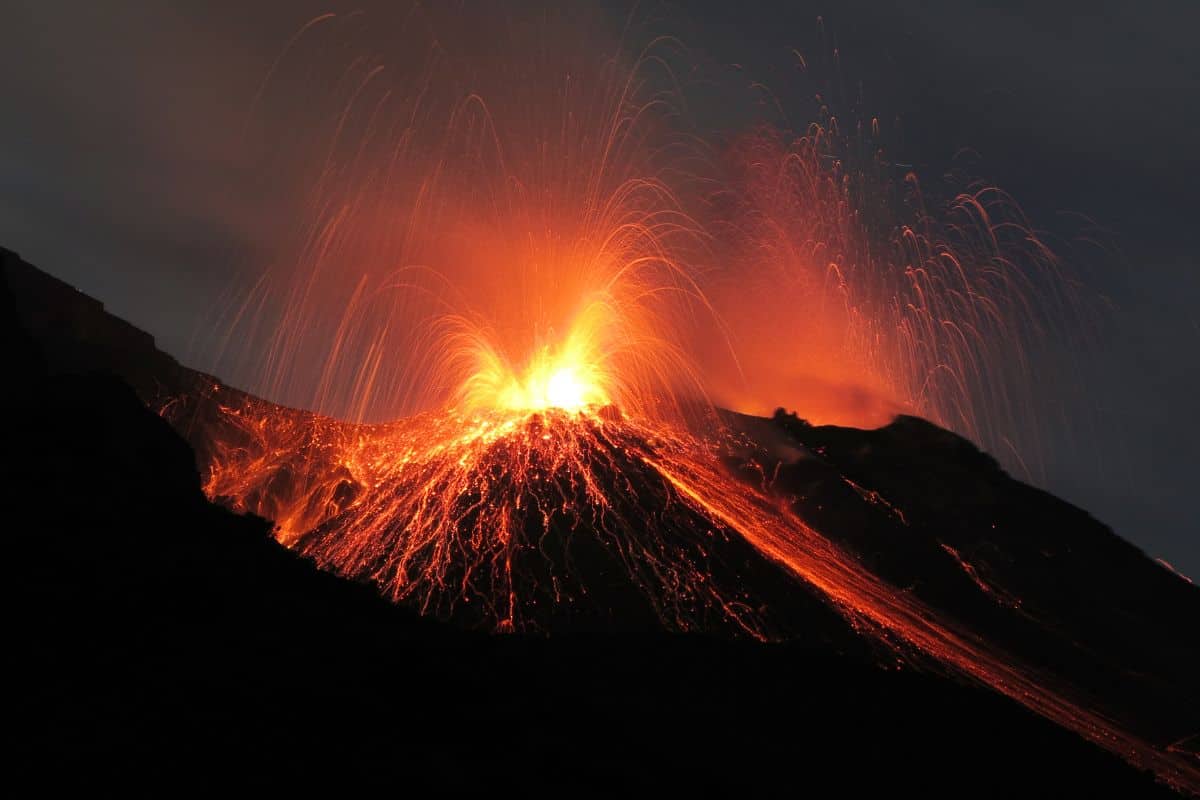In this striking nighttime image, we see a dramatic volcanic eruption against a backdrop of a pitch-black night sky. The volcano, centered within a wide-angled vertical frame, features a jagged and shadowy mountain silhouette that slopes down on both the left and right sides, with the middle section appearing relatively flat but rugged. From the top center of this jagged portion, vibrant red and orange flames erupt fiercely, arching upward before cascading back down, creating an effect reminiscent of a fiery fireworks display. Reddish-orange lava streams down the mountainside, adding a vivid contrast to the otherwise dark scene. The mountain itself is shrouded in shadows, merging almost seamlessly with the dark earth in the foreground, emphasizing the high, left-sloping curve of the mountain which then flattens in the center before descending sharply to the right. The dark sky above completes this powerful and awe-inspiring image of nature's raw, untamed energy.